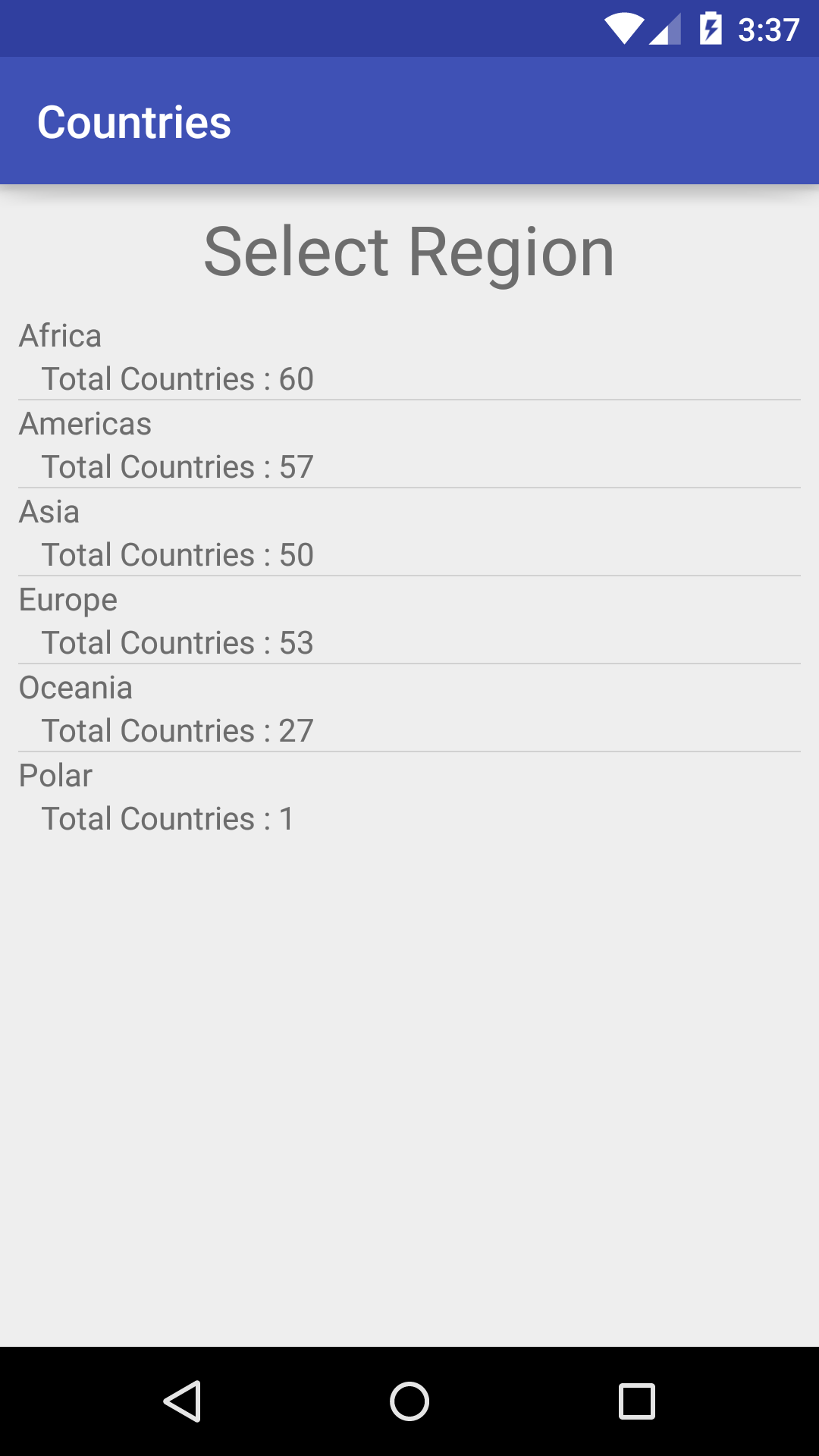Captured on a cell phone, this image displays a screen with several distinct elements. At the top, the status bar shows a fully charged battery icon with a lightning bolt, indicating that the device is plugged in and charging. The time is prominently displayed as 3:37, with a strong Wi-Fi connection also visible alongside it.

Below the status bar, a blue rectangular header reads "Countries." Directly beneath this, within a gray rectangular box, the text "Select Region" is prominently featured. The screen goes on to list various continents and their respective total number of countries: 
- Africa: 60 countries
- Americas: 57 countries
- Asia: 50 countries
- Europe: 53 countries
- Oceania: 27 countries
- Poplar (sic, possibly meant to be Popular): 1 country

The list extends towards the bottom of the screen, where an empty gray area provides no additional information, just a continuation of the background. Finally, at the very bottom, a black navigation bar spans from left to right, containing three icons: a white-tipped triangle (likely the Back button), a circle (Home button), and a square (Overview/Recent apps button).